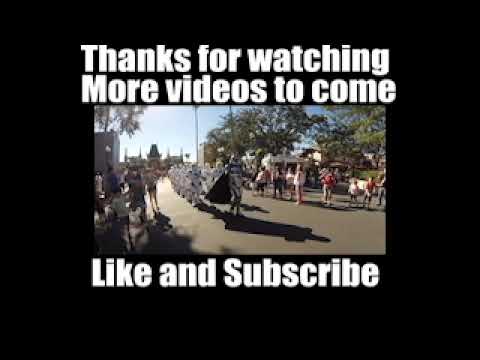A square image predominantly features a solid black background with a small horizontally aligned rectangle at the center. Inside this small central image, there is a giant statue of Woody, the main character from Toy Story, positioned in what appears to be an amusement park or playground setting. Woody, dressed in his recognizable cowboy hat and yellow outfit, is seated on a blue circular base. Surrounding this focal point, you can see a sidewalk, several buildings, and a tree. Additionally, there are giant children's blocks to the left of Woody, adding to the playground atmosphere. At the top of this inner image, in white text, it reads, "Thanks for watching, more videos to come." Below it, also in white text, it says, "like and subscribe." The rest of the square image remains a plain black, with a narrow strip of video artifacts running down the right edge, suggesting the image is a still captured from a video at varying resolutions.